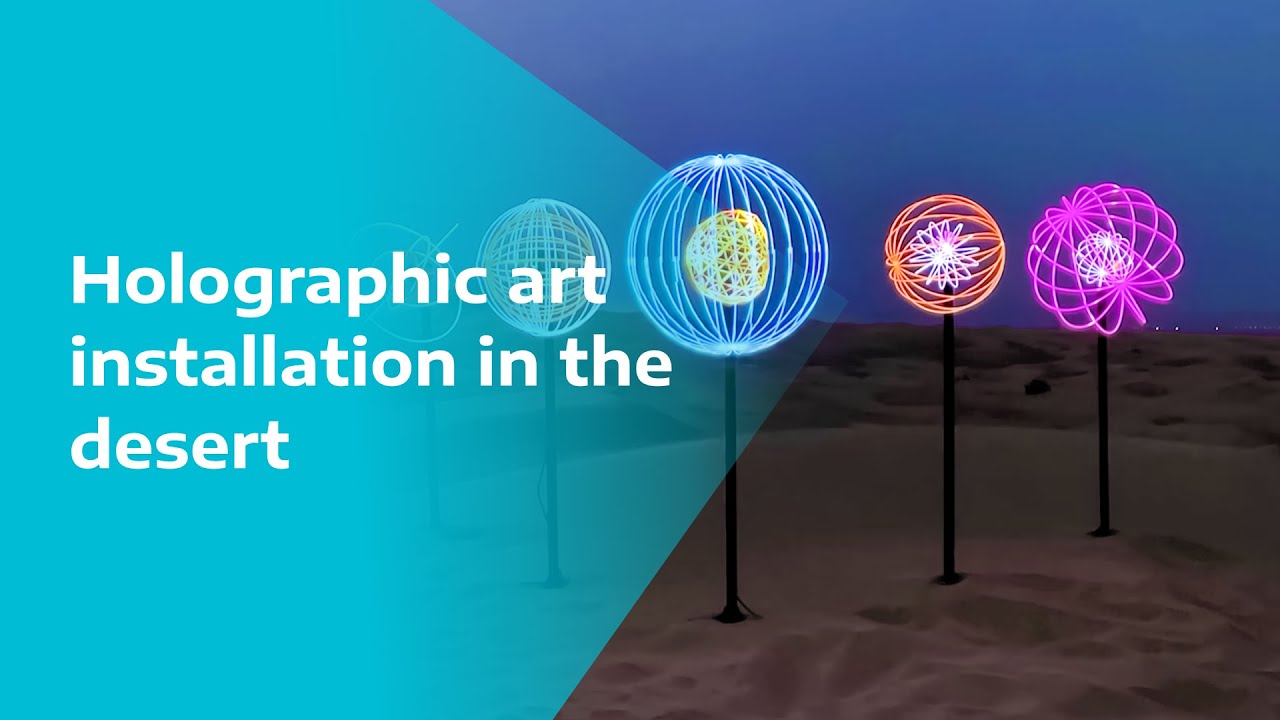This advertisement banner for an art exhibit showcases a striking holographic art installation set against a vast, sandy desert landscape. The rectangular banner features a semi-transparent light blue pentagonal overlay on the left side, with a prominent white text reading "Holographic Art Installation in the Desert," pointing toward the right. The right side of the banner, along with part of the left, depicts an array of black poles anchored in the white sand dunes. Each of these poles supports a glowing, neon-lit sphere. These luminous spheres are intricate, featuring various geometric designs crafted from LED lights, giving the impression of holographic structures made from radiant beams. The spheres display different colors: from right to left, the farthest right has magenta and white lights, followed by an orange and white sphere, and then a light blue with an orange center. Two further spheres are partially obscured by the pentagonal graphic but exhibit a light blue with yellow and an indistinct final color. The installation stands out starkly in the empty desert night, with distant lights on the horizon suggesting far-off buildings or vehicles.